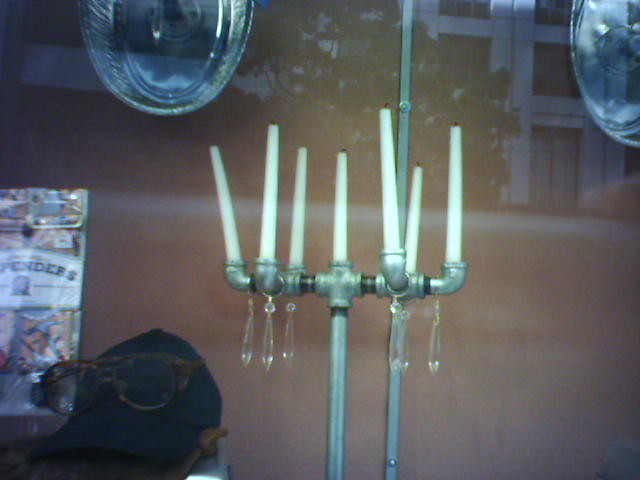This image captures an industrial-style, makeshift menorah crafted from steel piping, likely an art piece displayed behind glass, possibly in an antique store. The structure features two vertical pipes on either side connected to a central pipe fitting with three openings; one on top and two on the sides. The central fitting and side pipes hold a total of seven long white candles with visible black wicks. These candles are positioned in upturned piping elbows, creating a symmetrical arrangement with three candles on each side and one in the central top opening. Hanging from the horizontally running pipes are teardrop-shaped crystal ornaments, adding a touch of elegance to the otherwise industrial look. The background reveals a brown wall with two oval objects that resemble dishes. To the left, you can also see a package with a white banner, and in the lower-left corner, the head of a person wearing a blue baseball cap backwards with glasses resting on the bill.